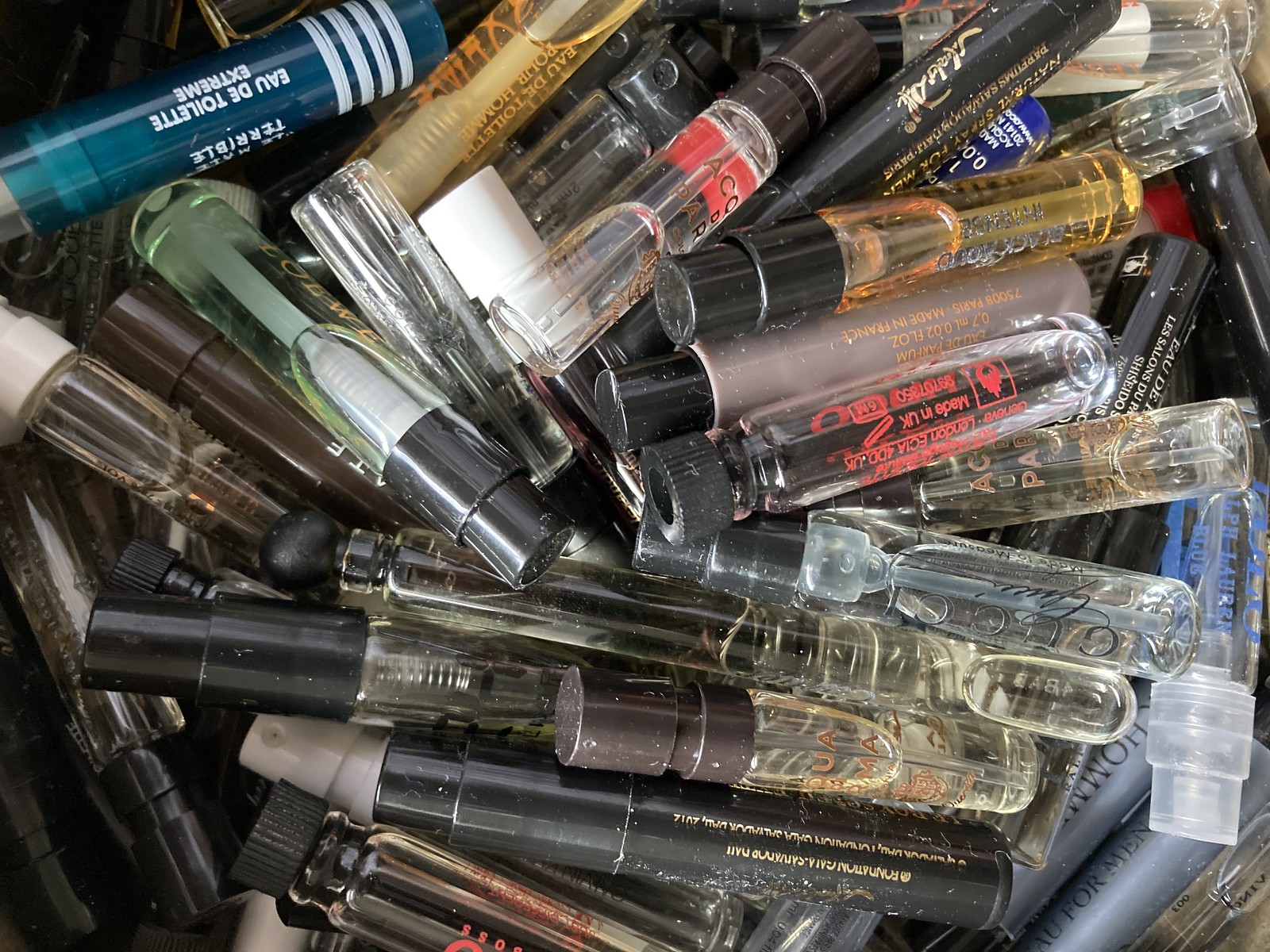The image presents a chaotic collection of 15 to 20 vials, each one marred with specks of dust, dirt, and skin flakes. These small, mostly translucent vials are intermixed with a handful featuring black or silver lids. Many appear to contain residual oils or liquids. The vials display a mix of squirt sprayers and screw-top lids, akin to those used with eyedroppers. An outlier among them, a single blue vial stands out. The text on all the vials is reversed, making it challenging to read since the image is upside down. The vials are haphazardly piled together, suggesting someone is discarding a collection of old and probably expired perfume samples. Many of the labels mention "eau de toilette," hinting at their original usage. These sample-sized vials, no larger than a middle finger in height and roughly a dime in diameter, create an impression of disarray and neglect, indicative of expired and potentially malodorous contents ready for disposal.